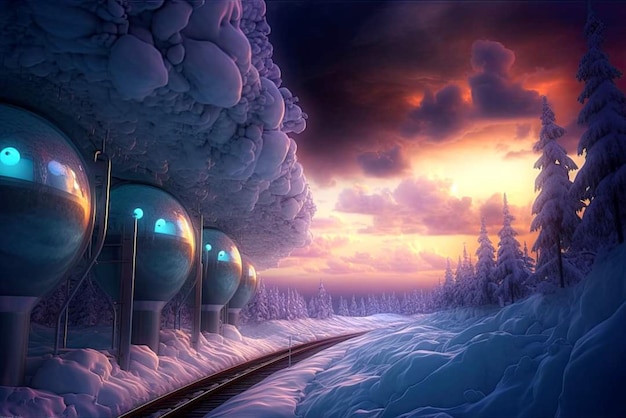In this AI-generated, futuristic image, a snowy landscape is illuminated by a stunning sunset, casting a yellowish-orange and red glow across the sky. The scene is bathed in shades of purple and blue, giving it an otherworldly atmosphere. A road or railroad track, dark and winding slightly to the right, cuts through the center of the landscape, surrounded by snow-covered evergreen trees.

On the upper left side, an anomalous, gravel-like purple cloud with bubble-like protrusions, resembling giant foam, adds to the surreal nature of the image. Below this peculiar cloud, four large, futuristic buildings stand out. These structures, resembling light bulbs or upside-down beakers, have a glass-like, see-through quality, with blue and indigo lights emanating from them. The delicate interplay of colors and the imaginative elements in this scene highlight its AI origins, blending a serene wintery setting with fantastical, sci-fi architecture.